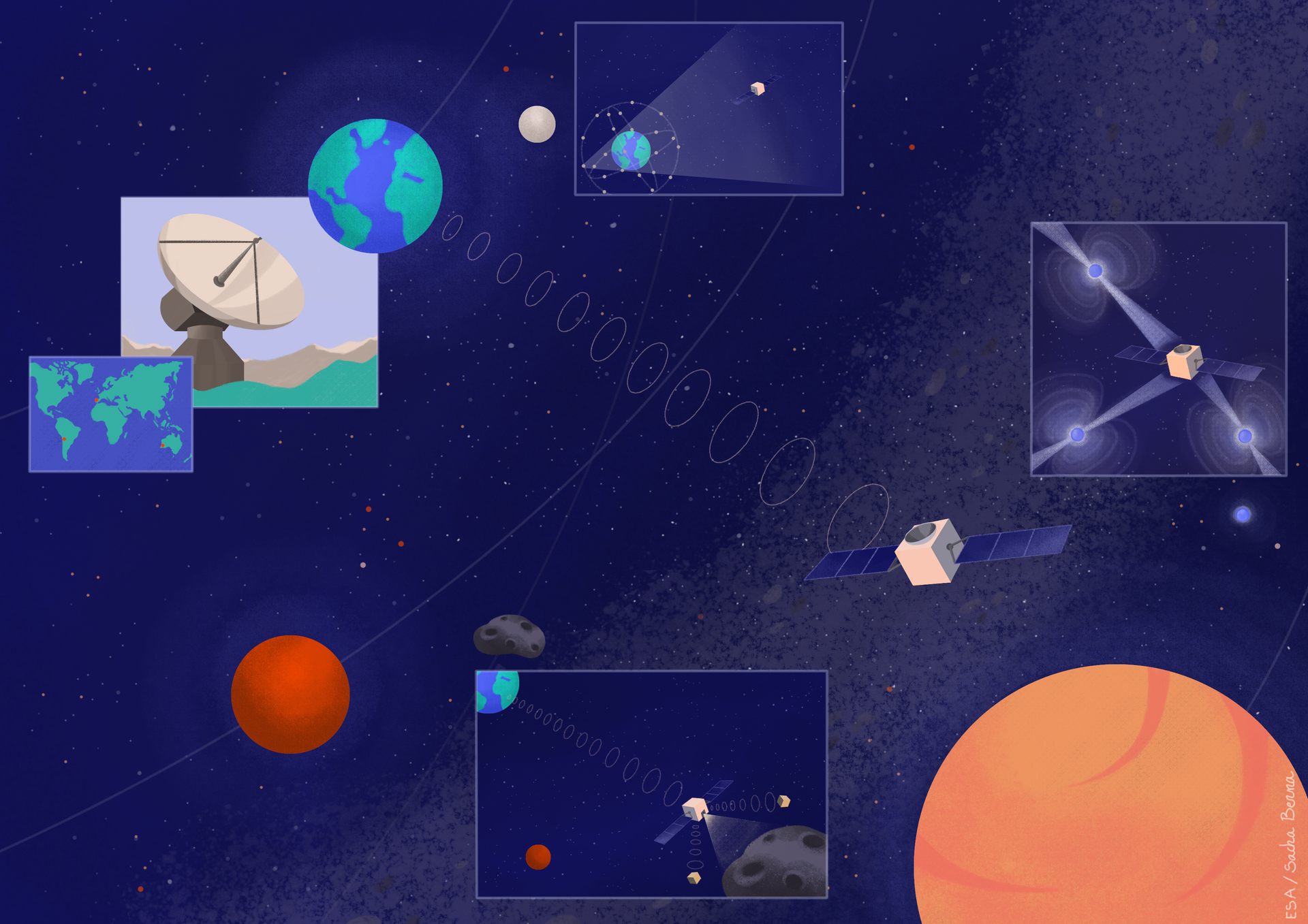This detailed graphic art piece features a rectangular image approximately five to six inches wide and four inches high, depicting a cosmic scene. The primary background is a dark blue, punctuated with specks of red and white, creating a starry night sky effect. A prominent one-inch wide stream of light gray debris sweeps from the upper right corner down toward the center, adding dynamic movement to the composition.

In the lower right corner, a large orange planet with tire-like stripes is partially visible, creating a striking contrast against the dark backdrop. Above this, an inset square displays an up-close graphic depiction of a satellite, complete with radiating beams. To the left of this, another satellite image is depicted with rings extending toward the upper left corner, culminating in a small globe representing Earth.

Adjacent to the satellite on the left is an image of the global map, showing different continents in detail. A thin white line starts from the lower left corner, rising upward, intersecting with a red circle that designates another planet. Nearby, a small black meteor is included, adding to the interstellar narrative.

One notable feature is a smaller inset that replicates the entire composition, offering a meta-view of the same graphic elements: Earth at the upper left, the satellite in the center, and a meteor and red planet to the left. Additionally, at the top center, a moon-like body is depicted, reinforcing the celestial theme. To the right of this is another boxed image of Earth, flanked by geometric shapes and another satellite, providing a sense of intricate cosmic connectivity.

Throughout the composition, various planetary bodies are depicted, including an ochre-hued cube situated prominently among the planets, adding an abstract, artistic touch to this detailed vision of space.